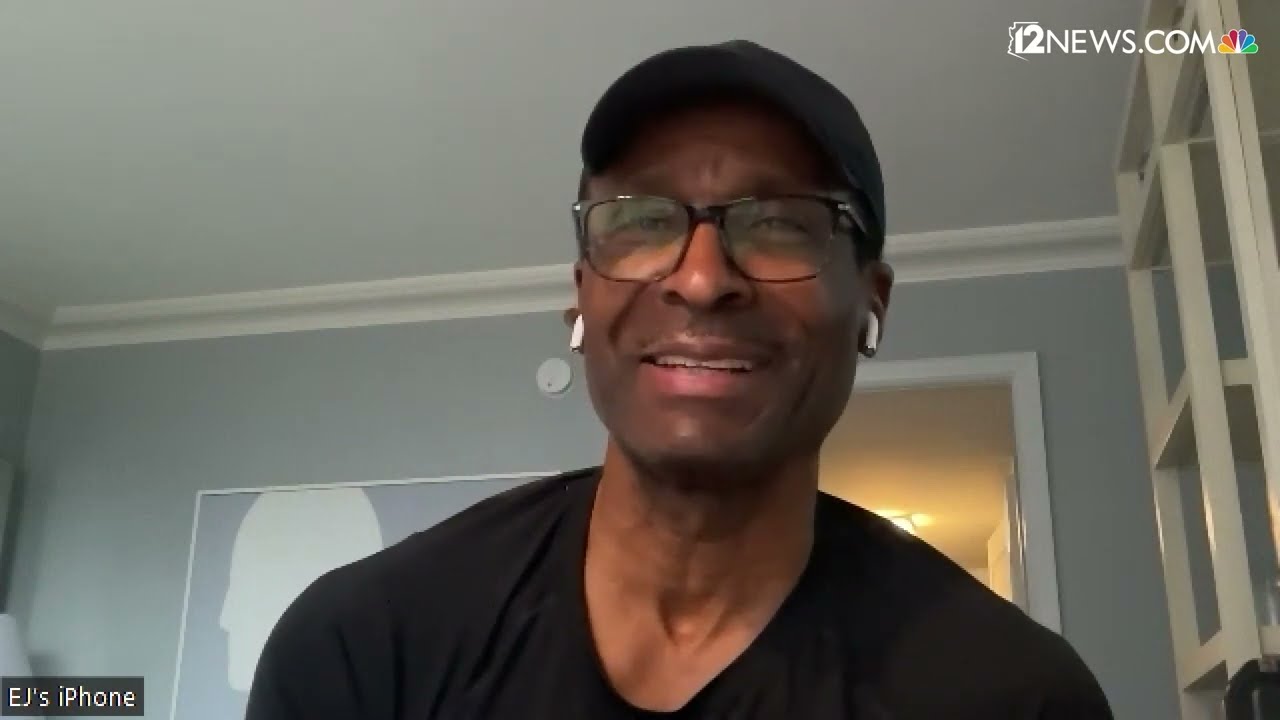The image is a detailed still from a news interview conducted over a video call, showcasing a black man, appearing to be around 40 years old, seated in front of a computer and facing a webcam. He is wearing a black baseball cap, brown-rimmed glasses, a black T-shirt, and white AirPods in his ears. His facial expression shows his eyes slightly closed and a partial smile, indicative of him possibly speaking during the call. In the background, the walls are painted a bluish-gray color with a white ceiling and white molding. The room includes white shelves to his right. Notably, at the bottom left corner of the image, there's a small opaque gray box with the text "EJ's iPhone," while the top right corner features the text "12 News" alongside the CNBC logo, indicated by the NBC peacock symbol.